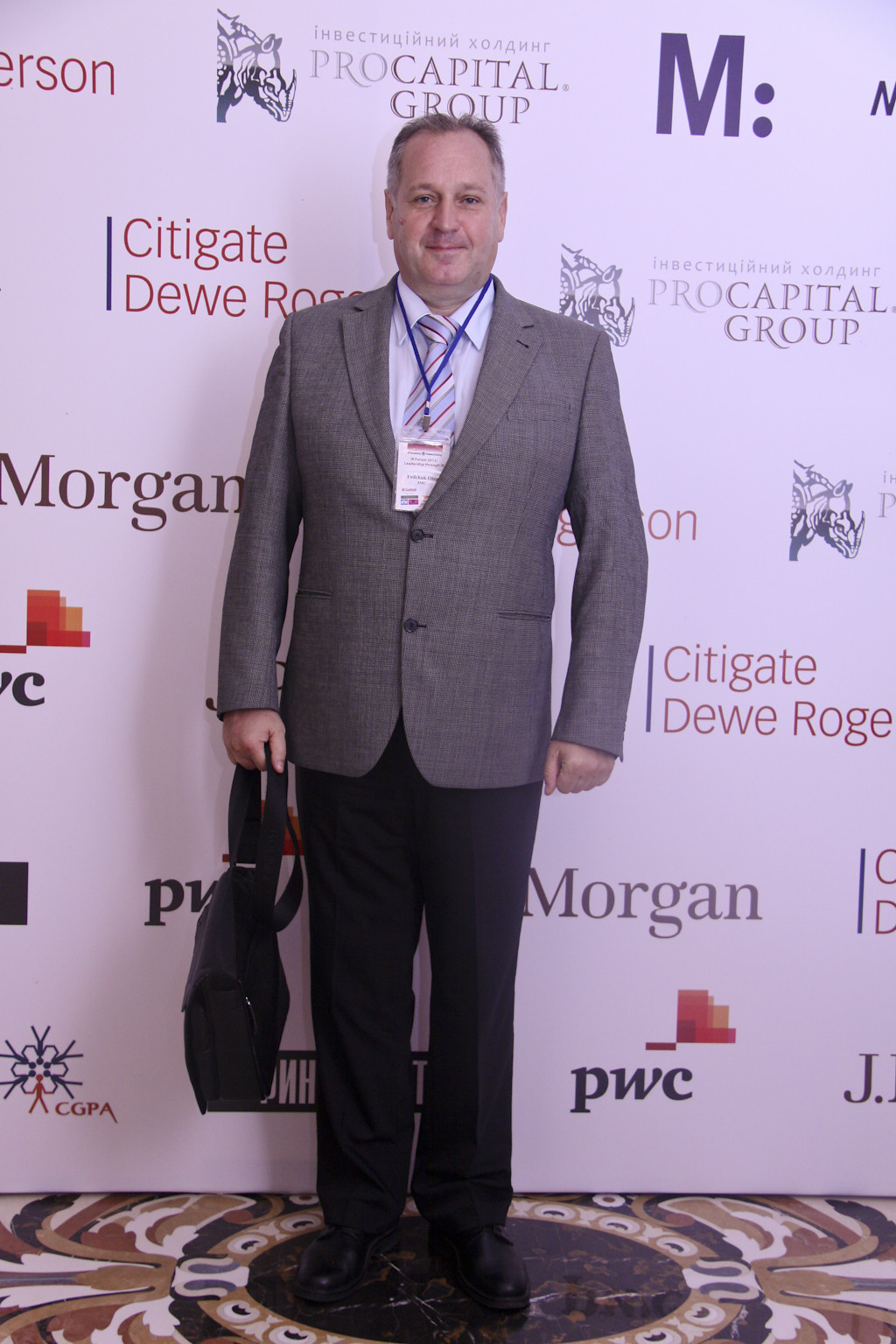In the image, a man stands directly in the center against a backdrop adorned with multiple logos, suggesting a formal event setting indoors. The backdrop features logos from various companies including Pro Capital Group, CityGate, Morgan, PWC, and CGPA. 

The man is dressed in a gray jacket paired with a light blue shirt, a blue, red, and white striped tie, and dark pants. He wears dark shoes and a blue lanyard with a badge around his neck. His right hand holds a bag, and his hands rest at his sides. His dark hair shows a touch of gray on the sides. The floor beneath him has a patterned design that appears painted or intricately detailed, incorporating colors like white, red, blue, black, purple, orange, yellow, brown, and tan.

The detailed attire of the man and the specific positioning of logos on the backdrop, alongside the diverse color patterns on the floor, collectively contribute to the formal and organized atmosphere of the scene.